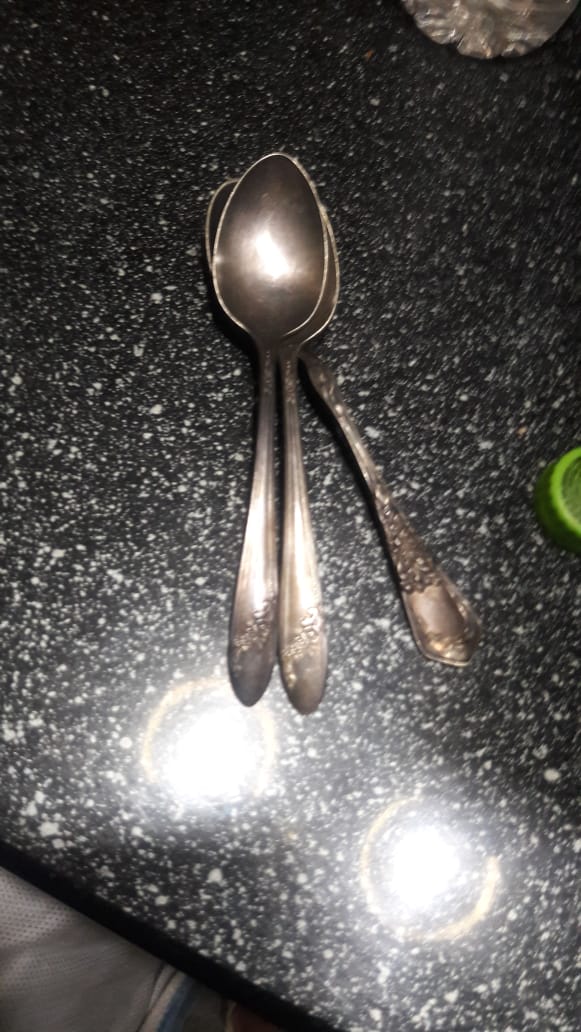This photo, seemingly taken with an older phone camera, features three silver spoons stacked on their bowls while their handles fan out slightly. The spoons have decorative engravings, suggesting they are fairly old, with the bottom spoon showcasing a different design from the other two. They rest upon a predominantly black marble countertop that is speckled with white. Reflections of two overhead lights are visible on the countertop, enhancing the detail of the scene. In the upper right corner, a sliver of what appears to be a plastic water bottle is visible, with the edge of a green cap partially cut off. The bottom left corner shows a bit of unidentified white netting or cloth, potentially part of a larger object just outside the frame.